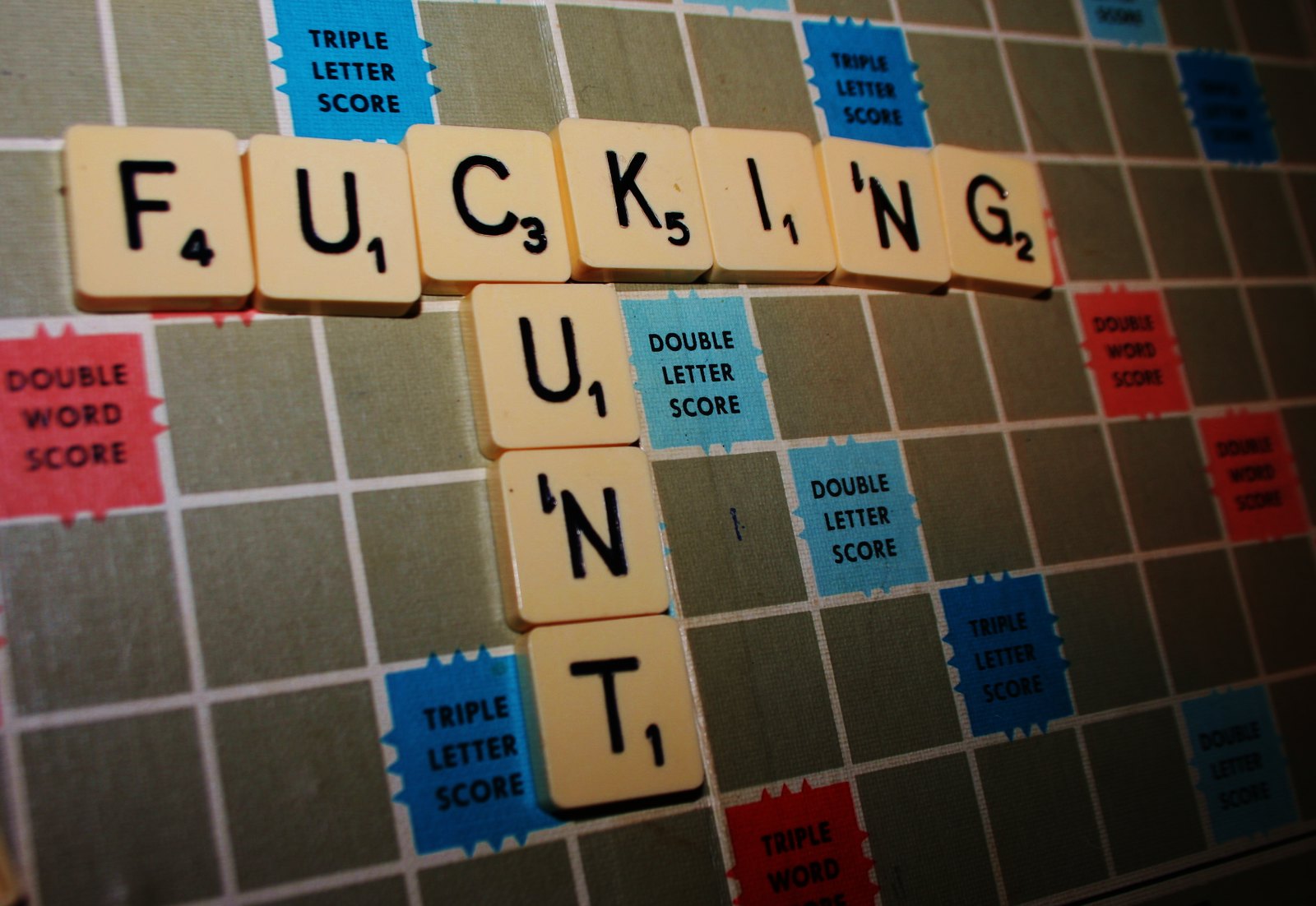The photograph displays a Scrabble board, arranged at an angle, showcasing a combination of highlighted squares of various colors and letters spelling out profanities. The board is a grayish-brown color, with prominent red, blue, and light blue squares representing different score multipliers: red signifies double word scores, light blue for double letter scores, and blue for triple letter scores. In the upper portion of the board, the letters are arranged to spell "FUCKING" horizontally, with each letter occupying individual squares. Vertically intersecting at the "C," the word "CUNT" is formed. The letters are detailed with their point values: F (4), U (1), C (3), K (5), I (1), N (1), G (2), with the intersecting C (3), U (1), N (1), and T (1). The words form a T-shape, leveraging both the board’s strategic multipliers and creating a stark visual of the crude language spelled out in the game setting.